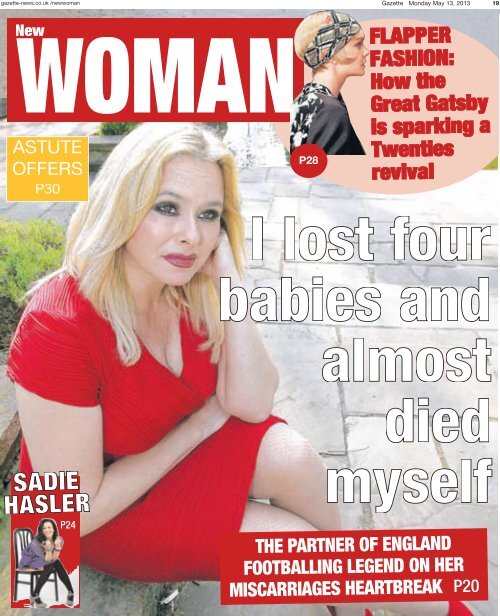The magazine cover of "New Woman" features a central image of a blonde woman in a red dress, sitting contemplatively on a stone bench with a sidewalk and grass in the background. At the top, the title "New Woman" is displayed in white font within a red rectangle. In the upper right corner, a smaller image depicts Carey Mulligan as Daisy Buchanan from "The Great Gatsby," adorned with a headscarf and flapper attire, next to the red-titled caption: "Flapper Fashion: How the Great Gatsby is Sparking a Twenties Revival". Below, in white font with a black border, the magazine highlights a personal story: "I lost four babies and almost died myself," further explaining "The Partner of England football legend on her miscarriage's heartbreak". Additional text near the bottom left notes an article by Sadie Hasler, with references to pages 28 and 30, including a snippet about "Astute Offers".